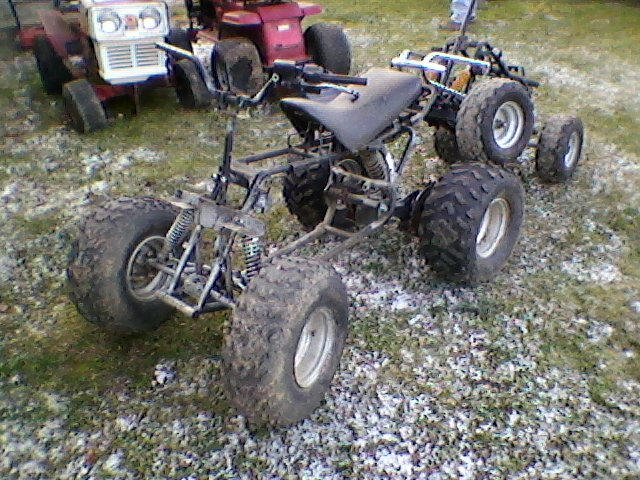The photograph captures a homemade ATV centered in the frame, situated on a grassy flat surface with scattered patches of snow or ice. The ATV features a basic, exposed frame without body panels, and is equipped with four chunky tires that are covered in grayish-brown dirt. A black saddle-like leather seat is positioned on top, and in front, there are black handlebars with integrated brakes, connected to the springs, suspensions, and steering mechanism for the front wheels. Attached to the rear is a trailer with an additional set of four tires, a black frame, and a yellow engine. The background reveals more vehicles of similar type, with two older, somewhat dilapidated red four-wheeled vehicles peeking into the upper left of the image, contributing to a slightly unkempt, trashy scene.